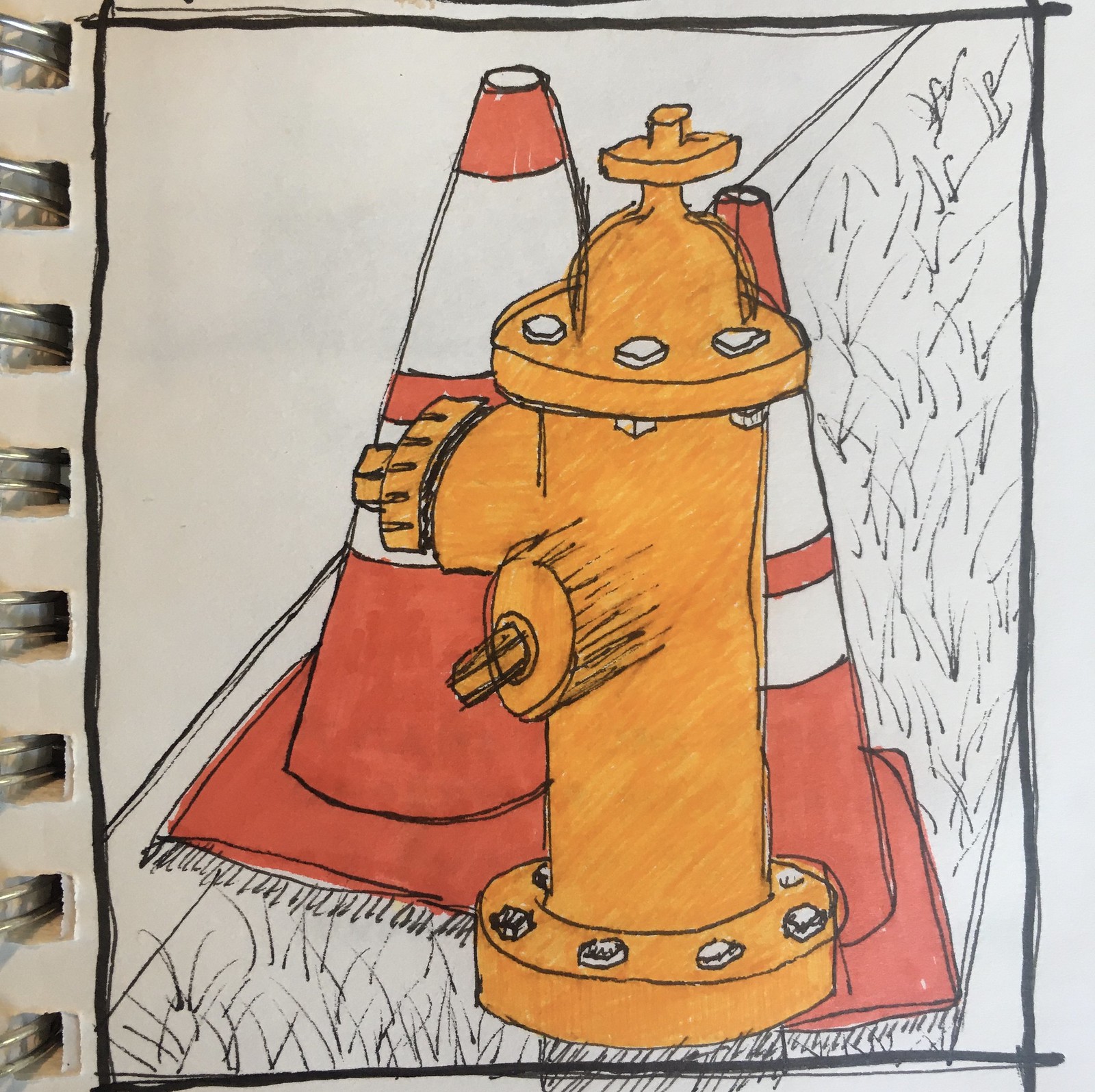This is a detailed hand-drawn artistic piece displayed in a spiral-bound sketchbook or art book. The drawing is enclosed within a thick black square border, created using colored pencils and possibly markers. At the center of the piece, there is a large, dull orange fire hydrant adorned with multiple white bolts and rivets. Sitting on a surface suggested by thin, curvy black lines indicating grass, the scene includes two traffic cones positioned behind the fire hydrant. These cones are colored in a dark orangish-red with distinctive white and orange stripes. The fire hydrant partially obstructs the view of the cones, which maintain a vertical stance with wide bases tapering to points as they extend upwards. The left side of the frame reveals the silver rings of the binder, with holes punched into the paper to accommodate them, indicating that it is part of a larger collection of sketches.